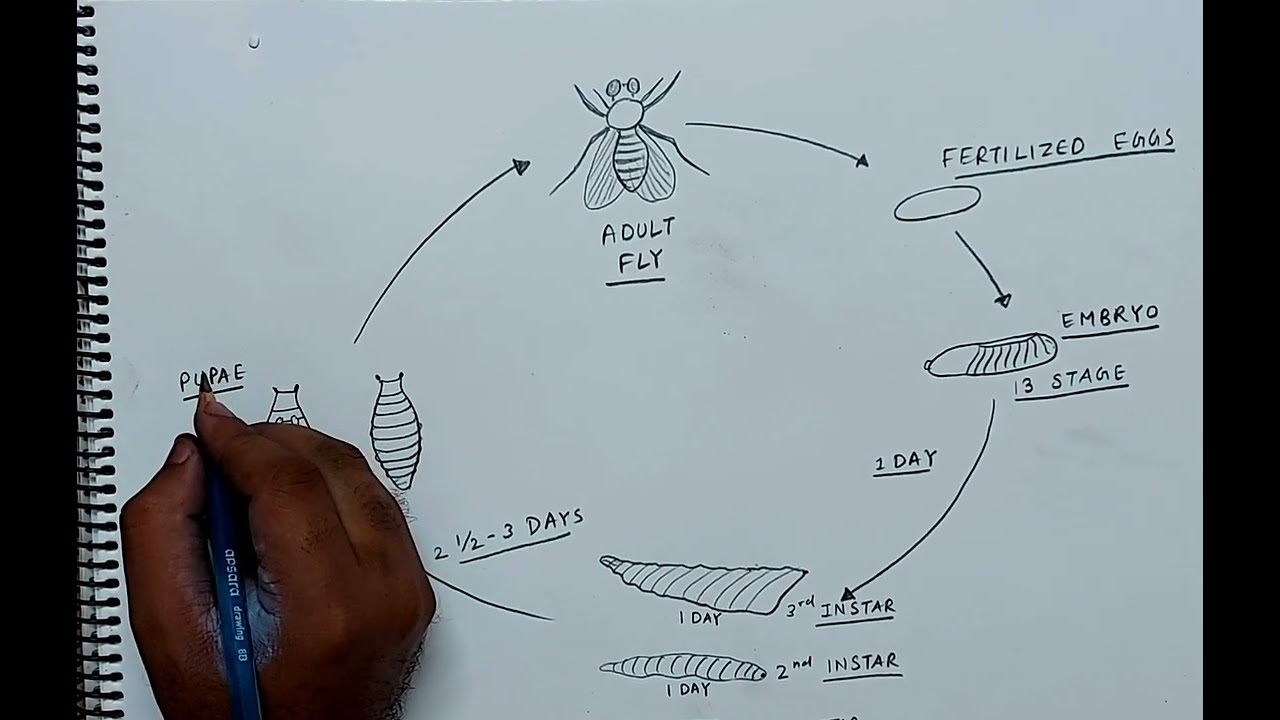In the image, a detailed drawing of the life cycle of a fly is depicted on a white notepad with a black spiral binder along the left edge. An Indian hand, positioned on the bottom left and holding a blue pencil, is actively engaged in the illustration, writing the word "pupae." The notepad features various stages of a fly's development, meticulously annotated with text and arrows. At the top center, a detailed drawing of an adult fly is labeled "adult fly." This is connected by an arrow to the right, leading to the text "fertilized eggs" and a corresponding drawing of eggs. Below this, the word "embryo" is written next to a sketch of an embryo. Further down, the development timeline continues with "one day" and drawings labeled "second instar" and "third instar," each connected by arrows and annotations. To the left, the text "two and a half to three days" is visible, indicating a later stage in development, likely the pupae. The entire image effectively showcases the sequential process of the fly's life cycle, from fertilized eggs to adulthood, through detailed hand-drawn illustrations and precise labels.